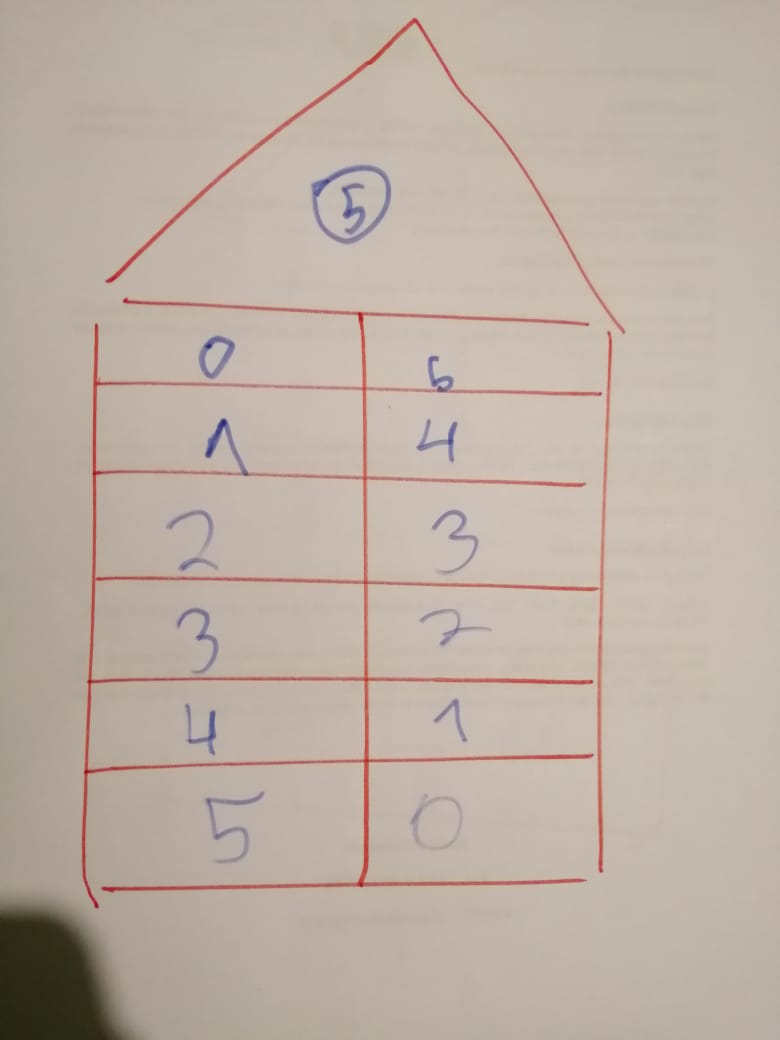The image depicts a stylized, hand-drawn representation of a house on a plain white sheet of paper. The house consists of a triangular roof and a square base, both prominently outlined in red. Inside the triangle, running vertically down its center, is a long red line. The square base also features several horizontal red lines dividing it into sections.

At the apex of the triangular roof, the number "5" is encircled in blue. This number sits on a red line that descends from the top of the triangle to its base. Below this, the square section features two columns of numbers, each written in blue. The first column lists the numbers "0," "7," "2," "3," "4," and "5," while the second column lists "6," "4," "3," "2," "7," and "0."

There is a subtle shadow visible in the left-hand corner of the white paper, lending a slight three-dimensional quality to the otherwise flat illustration.